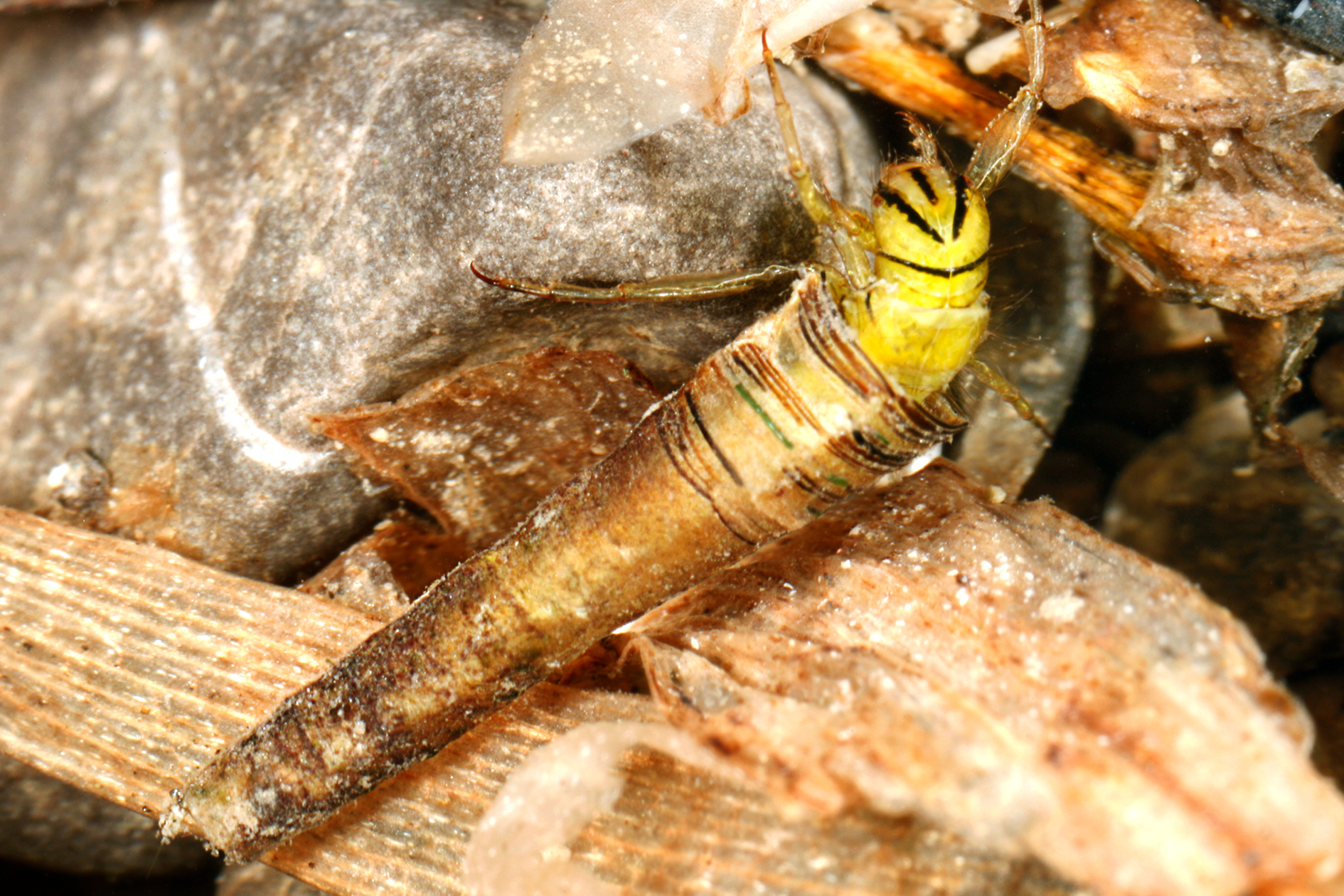This image is an outdoor close-up prominently featuring a large gray granite rock in the upper left-hand corner. Running across the bottom from one side to the other is a decaying piece of wood, resembling a thick board. Atop this weathered wood, which is sporadically adorned with leaves and spider webbing, rests an unusual and somewhat hideous insect. The insect is brown and shaped like an elongated cylinder or flashlight, wider at the top and narrower at the bottom. Its head is a striking yellow with three distinct black stripes, resembling eyebrows, and it sports two thin antennae that could be mistaken for horns. Emerging from an open, translucent cocoon or shell, the insect's legs are visible, suggesting that it might be in the process of emerging or resting upon the debris-covered wooden board.